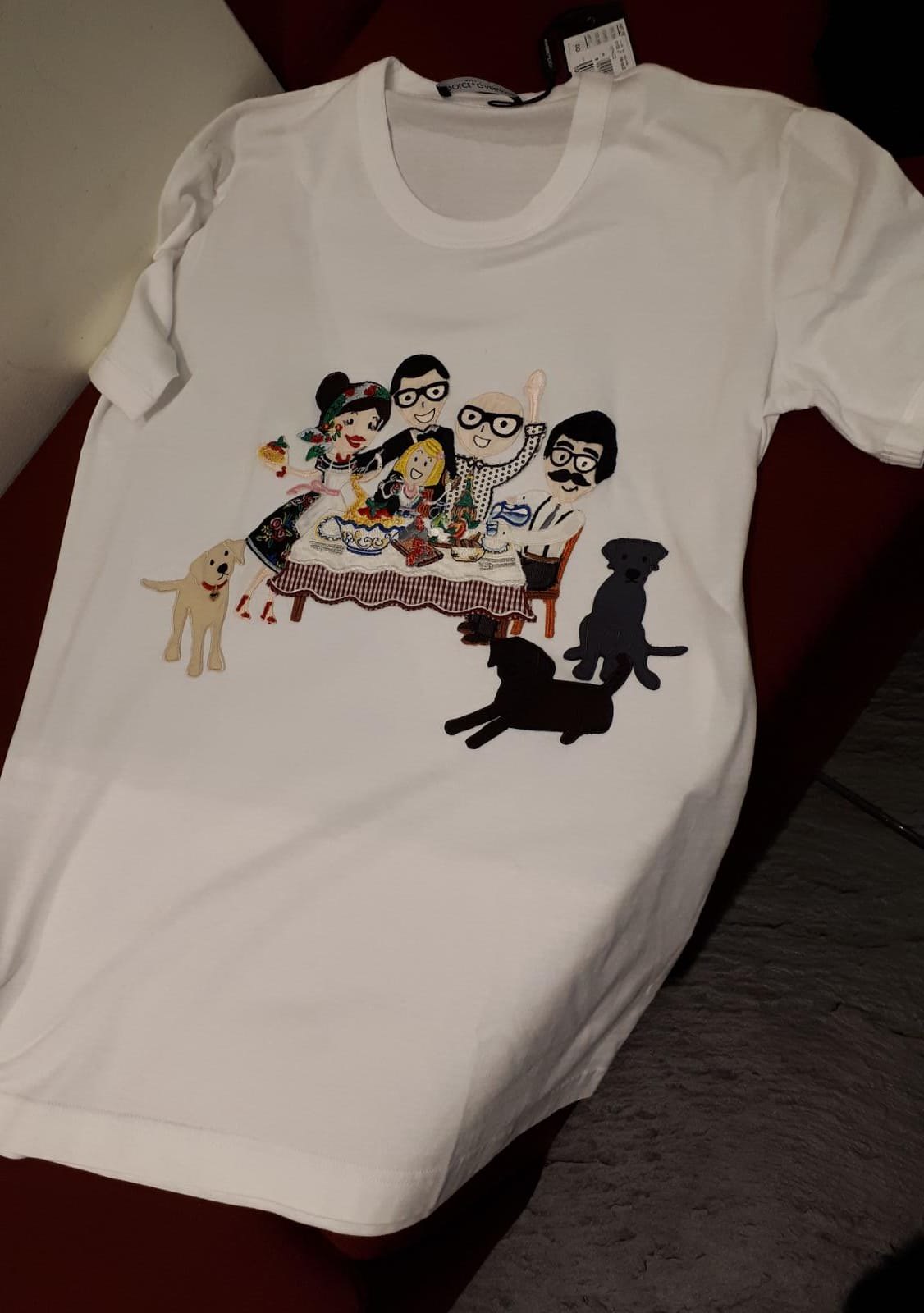The photograph features a white T-shirt meticulously spread out on what appears to be a bench. The bench rests upon a large gray tile floor, accentuated with black grout lines. This white T-shirt, with its crew neck collar and short sleeves, exudes a distinct rough texture. 

A price tag is visibly attached to the back of the T-shirt. The front showcases a vividly embroidered illustration depicting a heartwarming family scene. In the illustration, a family is gathered around a table covered with a white tablecloth adorned with a red checked border. Situated around the table's base are three dogs: a gray one sitting upright on the left, a dark one lying down in the middle, and a light-colored one standing to the right.

At the table, a woman with a scarf draped over her head is accompanied by three men and a little girl, adding a touch of charm and narrative to this detailed and textured T-shirt design.